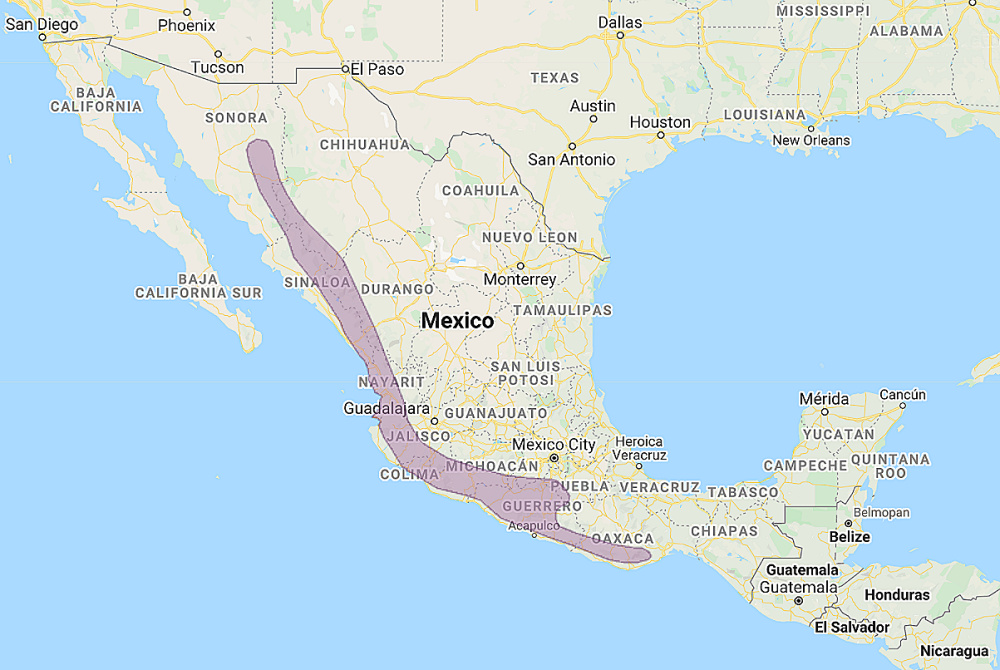The image shows a detailed Google Maps screenshot encompassing Mexico, with parts of the southern United States and northern Central America, including Guatemala, Honduras, and El Salvador, also visible. The focus is primarily on Mexico's center and west coast. A substantial portion of the west coast is highlighted in a semi-transparent, dull red color, suggesting the presence of a significant feature such as a weather pattern or geological formation. The highlighted area extends from the state of Sonora in the north, down to Oaxaca in the south, forming a long, continuous strip though not covering the entire coastline or spanning from border to border. Baja California is notably unaffected. The absence of additional context leaves the specific significance of this red-highlighted region open to interpretation.